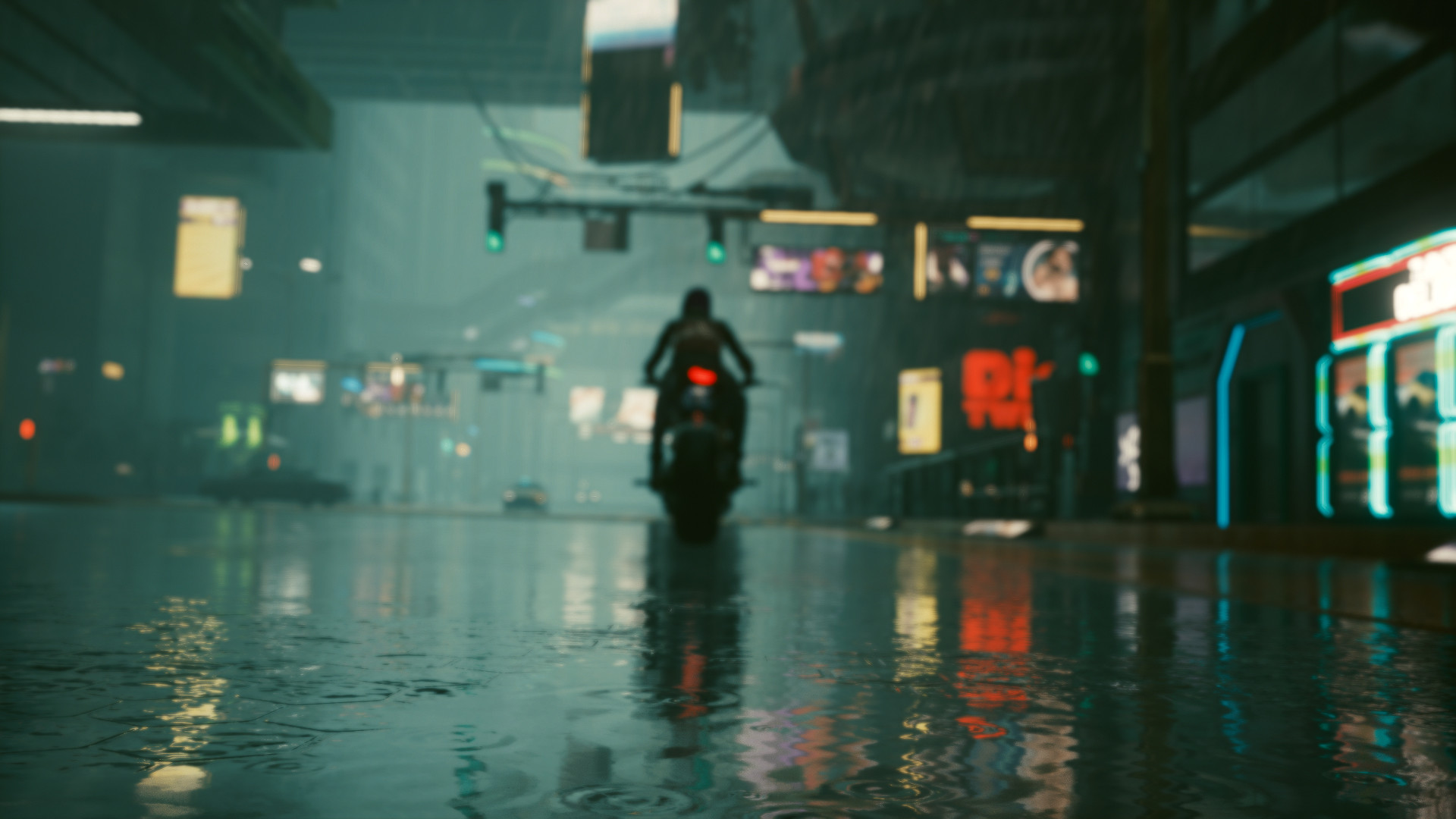This photograph captures a vibrant city street on a rainy night. The wet road gleams under the city lights, reflecting the multicolored brilliance from various sources. In the foreground, a motorcycle is stopped at a traffic signal, its red rear light piercing through the night. The stoplight above shows two green lights, indicating movement in other directions.  

Further along the street, a few other cars can be seen, their lights blending into the urban backdrop. To the right, a store illuminates the scene with green, red, and white lights glowing in its windows, adding to the colorful mosaic of the city night. In the distance, a brightly lit sign with red letters partially reads 'D', 'I', 'T', and 'W', offering a focal point among the numerous lights of buildings and street lamps.